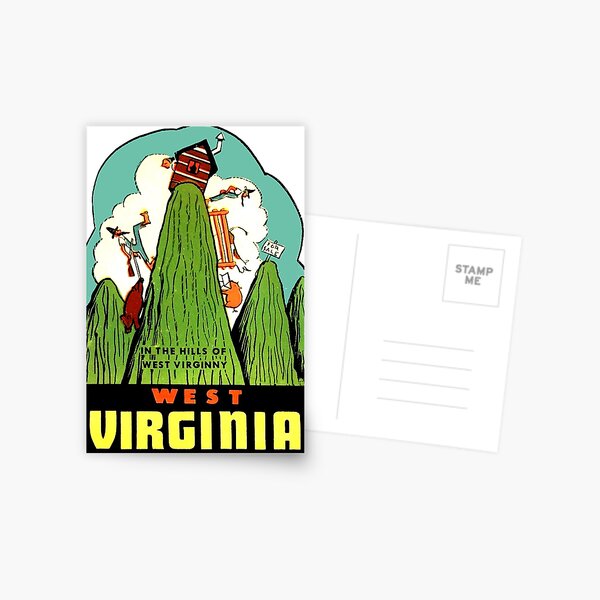The image depicts a single postcard set against a completely smooth white surface. The postcard showcases two sides. On one side, a stamp is placed on the left, covering part of the envelope. To the right, in the top corner, is a square indicating where stamps should be placed, labeled "stamp me." Below this, there are four lines allocated for the recipient's address.

On the other side of the postcard, the scene is set "In the hills of West Virginia," as indicated by text running across the central mountain with "West Virginia" written below in a black banner, "West" in red, and "Virginia" in yellow. This side features an intricate cartoon-style illustration of steep, green mountains. At the top of the central mountain is a quaint, red-and-white striped shack with a silver chimney. A character dressed in blue overalls, a white shirt, and a pointy hat – possibly a West Virginia mountaineer or farmer – is climbing the steep incline, pulling along a wild boar. Another similar figure rests on a bench on the right side of the mountain. The background illustrates a light blue sky with big, white puffy clouds, and additional details include a yellow fence with an orange and white cat perched on it, a scarecrow or another farmer figure by the fence, cows, pigs, and a bear near the shack. This whimsical and detailed scene captures the rural charm and rugged terrain of West Virginia.